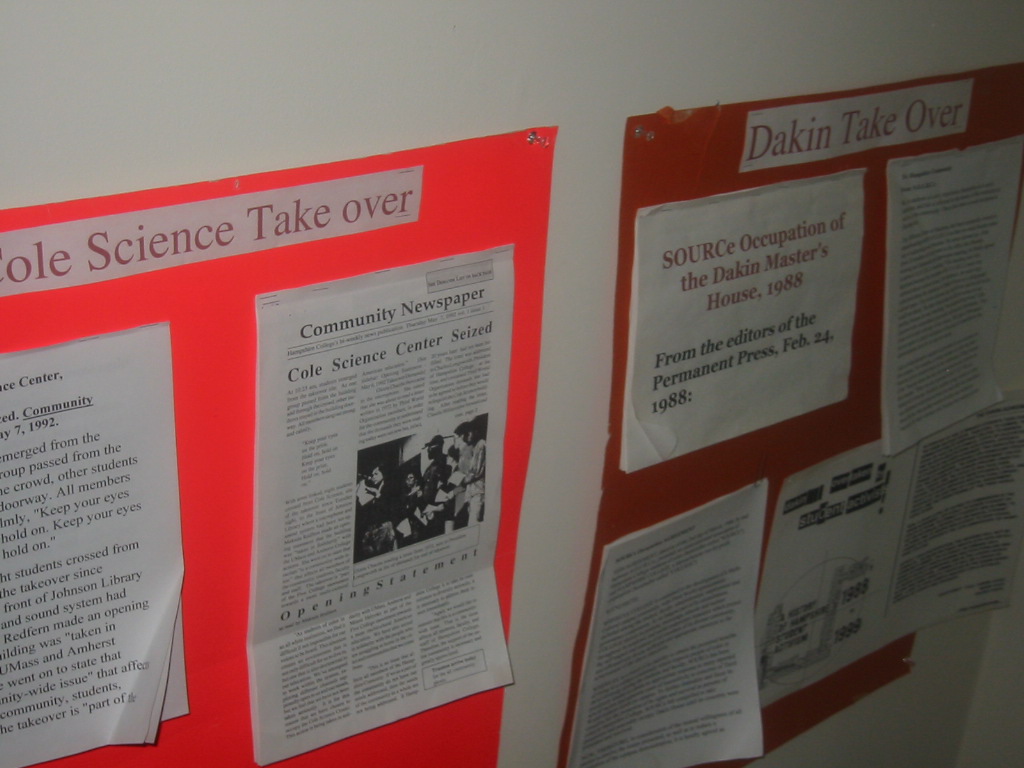This photograph captures a wall adorned with approximately seven pinned clippings, likely situated in a school or office environment. Dominating the scene are two prominent posters, one in a salmon hue and the other in dark orange, partially cut off on their respective sides. The salmon-colored poster on the left features clippings such as "Community Newspaper" and "Coal Science Center Seized," with visible dates like the 7th day of 1992. The dark orange poster on the right is titled "Dakin Takeover" and includes headlines like "Source Occupation of the Dakin Master's House, 1988" and "February 24, 1988, from the editors of the Permanent Press." This poster also features a piece of paper with a diagram and additional text at its top. Together, these clippings and posters offer a historical glimpse into significant events and publications from the late 1980s and early 1990s.